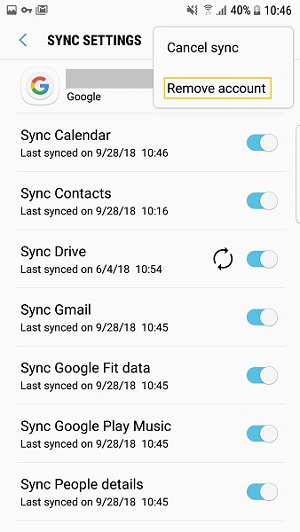The image displays a smartphone screen showing a website. The phone's interface indicates that the time is 10:46 AM, and the battery level is at 40%, with a stable internet connection. The sound settings appear to be muted, as suggested by an icon.

On the left side of the screen, three small icons are visible. The page is titled "Sync Settings." A white pop-up box on the right side of the screen features two options: "Cancel Sync" and "Remove Account," with the latter outlined in gold. Below these options, there is a gray bar labeled "Google," accompanied by Google's round, multicolored "G" logo.

The list below includes the following synchronization options, each with a toggle switch next to it:
- Sync Calendar
- Sync Contacts
- Sync Drive
- Sync Gmail
- Sync Google Fit data
- Sync Google Play Music
- Sync People details

The toggles are designed in such a way that when a sync option is enabled, the switch turns blue; when disabled, it appears as a light gray circle.

The entire scene confirms that the website is accessed from a phone, evident by the vertical orientation of the display and the proportions that fit a smartphone screen.